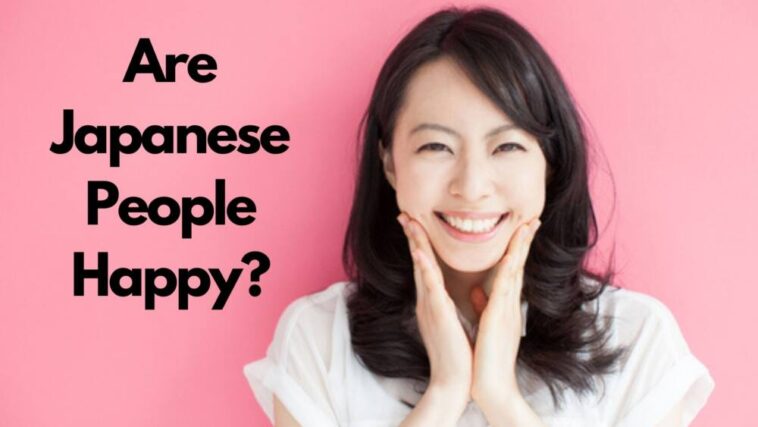The poster features a cheerful Japanese woman with long, dark brown hair, adorned with bangs swept to the left and a large curl at the bottom. She is dressed in a white blouse and stands against a brightly lit pink background. The left side of the poster displays bold black text arranged in four lines, reading "Are Japanese People Happy?" The woman, positioned to the right of the text, is beaming with joy, her eyes glowing and her big smile accentuating her happiness. She holds her cheeks with both hands, as if to emphasize her elation. The image, rectangular and wider than it is tall, juxtaposes the question with the woman's vivid expression, presenting an alluring, optimistic scene.